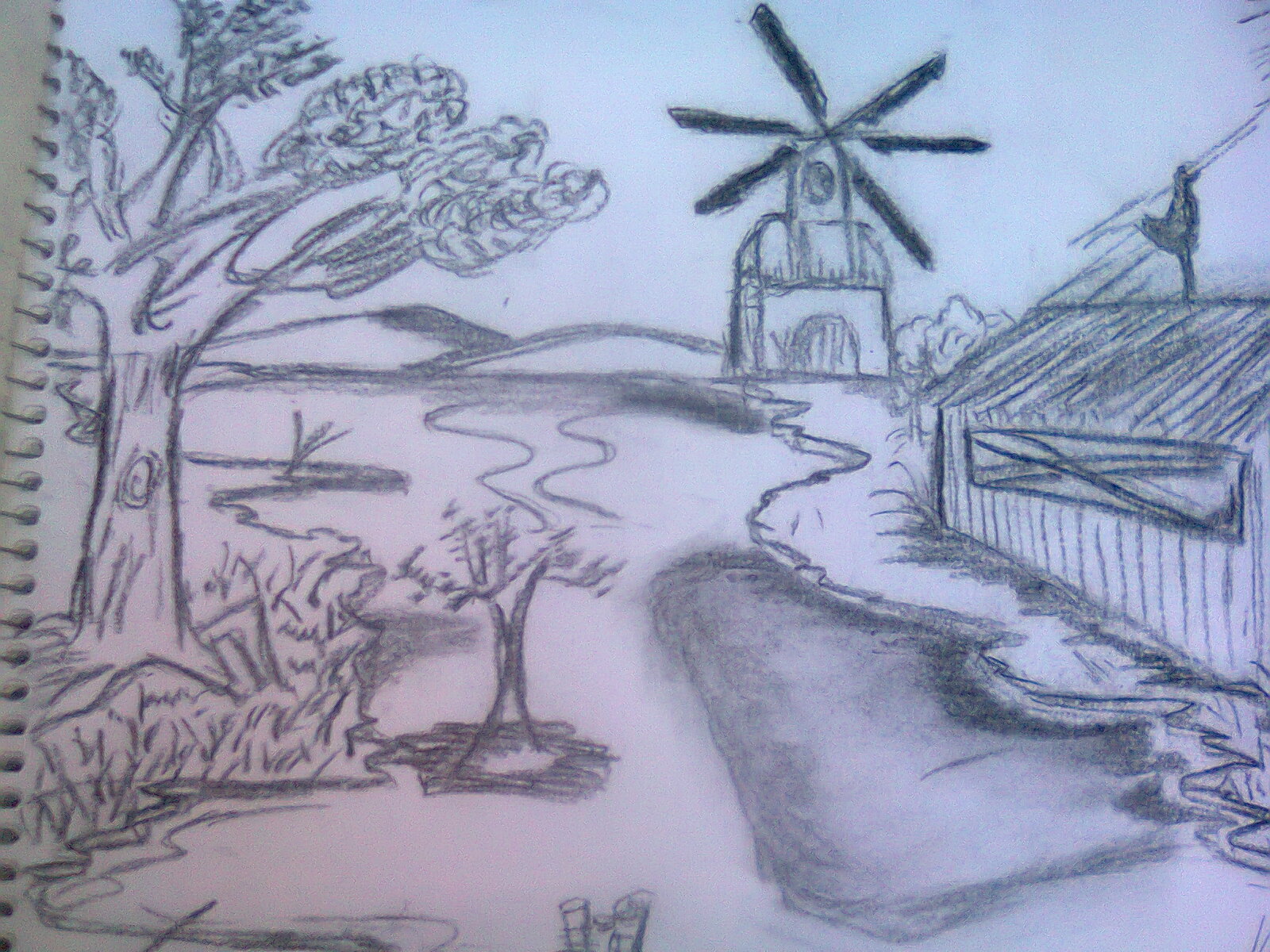This image showcases a meticulously detailed pencil sketch on plain white paper, set against the presence of a spiral-bound notebook, which is evident from the spiral binding seen along the left edge of the frame. The sketch depicts a serene creek or river scene enveloped in natural beauty. On the left side of the composition, a cluster of trees rises gracefully, their foliage providing a lush contrast to the scene. In the distance, softly undulating hills or low-sloped mountains create a tranquil backdrop.

Towards the right side of the frame, a windmill stands tall, partially obscured by the rolling hills. The water appears to originate from the direction of the windmill, meandering gracefully towards the foreground where a quaint shed or barn is positioned. Perched atop this structure is a charming rooster ornament, adding a whimsical touch to the composition.

In the lower left corner, beneath a prominent tree, patches of grass and a smaller tree are interspersed throughout a field, suggesting an area of greenery. Additionally, there is a shaded section in the bottom center-right of the image, which might represent a rock or more eroded terrain, further enhancing the natural diversity of the scene.